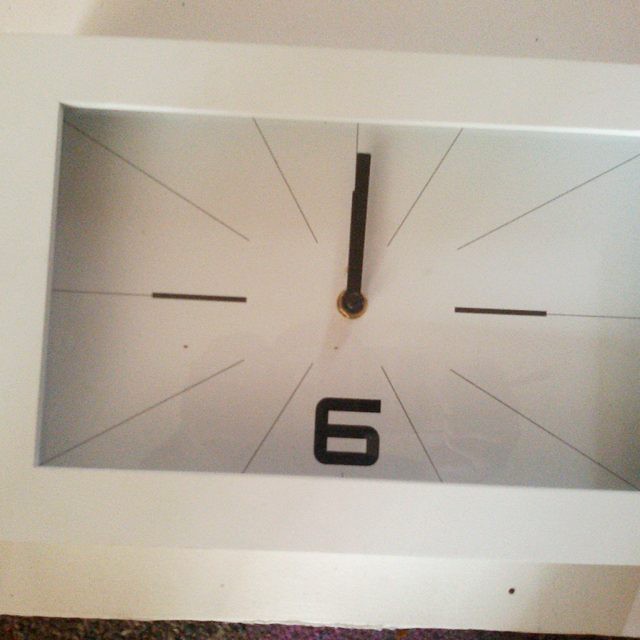A minimalist, rectangular white clock is captured in this photograph. The clock, which features a thick border that may be composed of wood, metal, or plastic, is elegantly designed with a stark, clean aesthetic. The most striking element on the clock face is a large black number six at the bottom, juxtaposed with the absence of other numbers, which are instead represented by slender black lines. Thicker black lines mark the positions where the numbers three and nine would traditionally be. The time shown is midnight, with bold, elongated hour and minute hands pointing straight up in a stick-like fashion. Intriguingly, the clock's reflective surface catches the silhouette of the photographer, adding a personal, shadowy presence to the image.